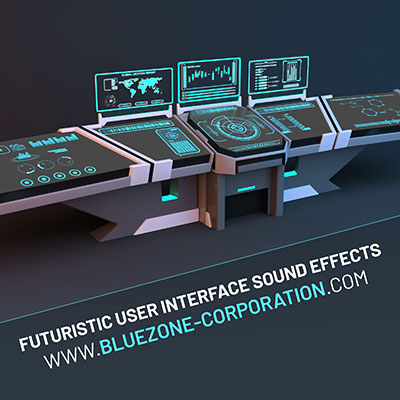This is a detailed, color drawing of a futuristic user interface, designed to evoke high-tech environments such as those found in a starship, submarine, or aerospace control room. The background is primarily black with subtle shades of gray, creating a stark contrast for the bright, light bluish-green elements that make up the intricate design. 

Dominating the scene is an array of at least five instrument panels and three monitors, all displaying different graphics and data. One monitor prominently shows a world map, another displays a large compass, and a third is filled with various graphs. 

The entire setup is reminiscent of a comprehensive control board, with the panels and monitors organized in a desk-like format that extends across the screen. These panels are of varied, non-rectangular shapes, adding to the futuristic aesthetic with their slanted and irregular forms.

At the bottom of the image, a line cuts across at an angle, below which bold white text reads "Futuristic User Interface Sound Effects" alongside the website URL "www.bluezonecorporation.com". Notably, "Bluezone Corporation" is distinguished in a light bluish-green hue, matching the color scheme of the interface graphics above.